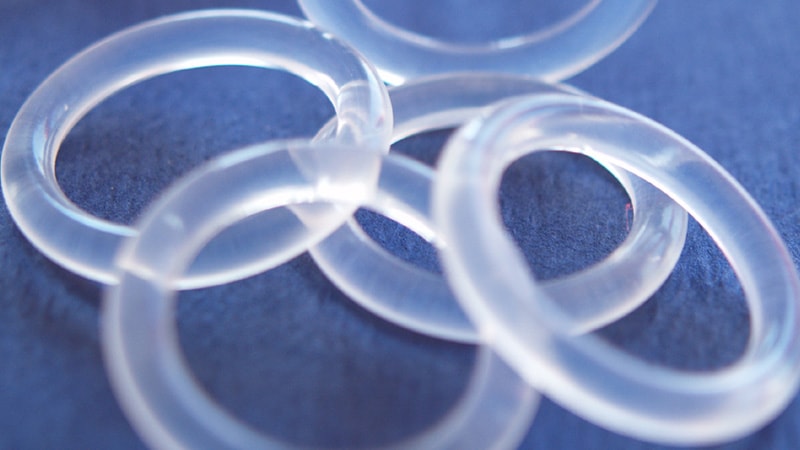This image features five clear, plastic rings arranged in a way that they overlap each other, creating a layered effect. The rings are approximately three to four inches in diameter and resemble the Olympic symbol, though all rings are transparent. The clarity allows light to shine through, making them appear opaque in some areas while remaining clear in others. This interplay of light adds a dynamic quality to the rings. The background is a blue, denim-like fabric, with visible threads providing texture and contrast to the smooth surface of the rings. The topmost ring is partially visible, emphasizing the overlapping arrangement.